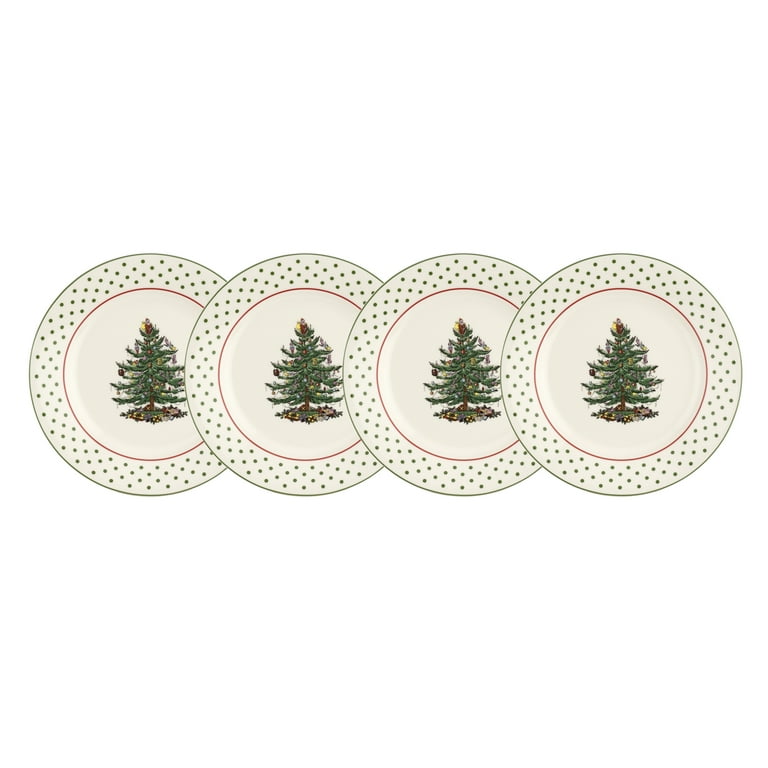The image showcases four Spode Christmas plates arranged on a pure white background. Each plate, overlapping slightly with its neighbor, features similar intricate designs. Centered within each cream-colored, off-white plate is a decorated green Christmas tree adorned with vintage ornaments and candle-like decorations, topped possibly by a Santa figure, and surrounded by what appears to be a tree skirt. Encircling the tree, a red line creates a striking contrast, beyond which the border is sprinkled with small green polka dots. The design is completed with a thin green line at the very edge of each plate.